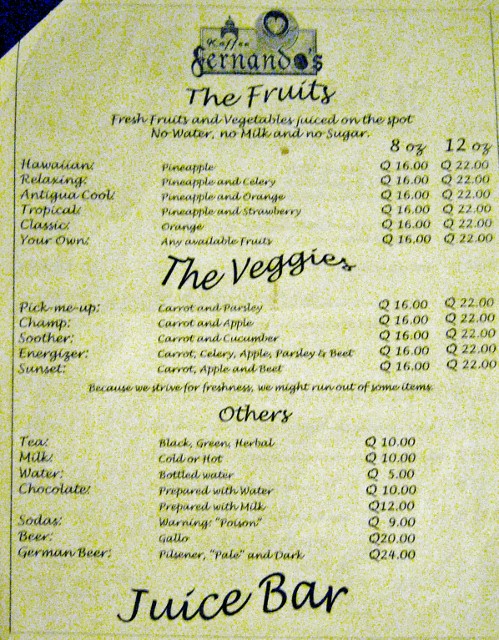The image depicts a restaurant menu with a vintage design, resembling a juice bar's offerings. The menu's background is a beige color with yellow splotches scattered throughout. The text is in black, making it somewhat difficult to read. The name on the menu appears to be "Keffin Fernandos," with an old-world font style, and notably, the 'O' in "Fernandos" is completely blacked out. 

At the top of the menu, there are two images, though their specifics are unclear. The menu highlights its focus on fresh fruits and vegetables, explicitly stating that the juices are made on the spot without added water, milk, or sugar.

The fruit juice section includes the following options:
- **Hawaiian**: Pineapple
- **Relaxing**: Pineapple and celery
- **Antiqua Cool**: Pineapple and orange
- **Tropical**: Pineapple and strawberry
- **Classical**: Orange
- **Custom**: Any available fruits of your choice

Pricing for the fruit juices:
- 8 ounces: $16
- 12 ounces: $22

The vegetable juice section offers:
- **Sunset**: Carrot and parsley
- **Energizer**: Carrot and apple
- **Soother**: Carrot and cucumber
- **Champ**: Carrot, celery, apple, parsley, and beet
- **Custom**: Carrot, apple, and beet

The prices for the vegetable juices are the same as the fruit juices, ranging from $16 to $22 depending on size.

The menu also mentions that due to the commitment to freshness, there may be times when certain items are unavailable. Other beverages listed include tea, milk, water, chocolate, soda, beer, and German beer.